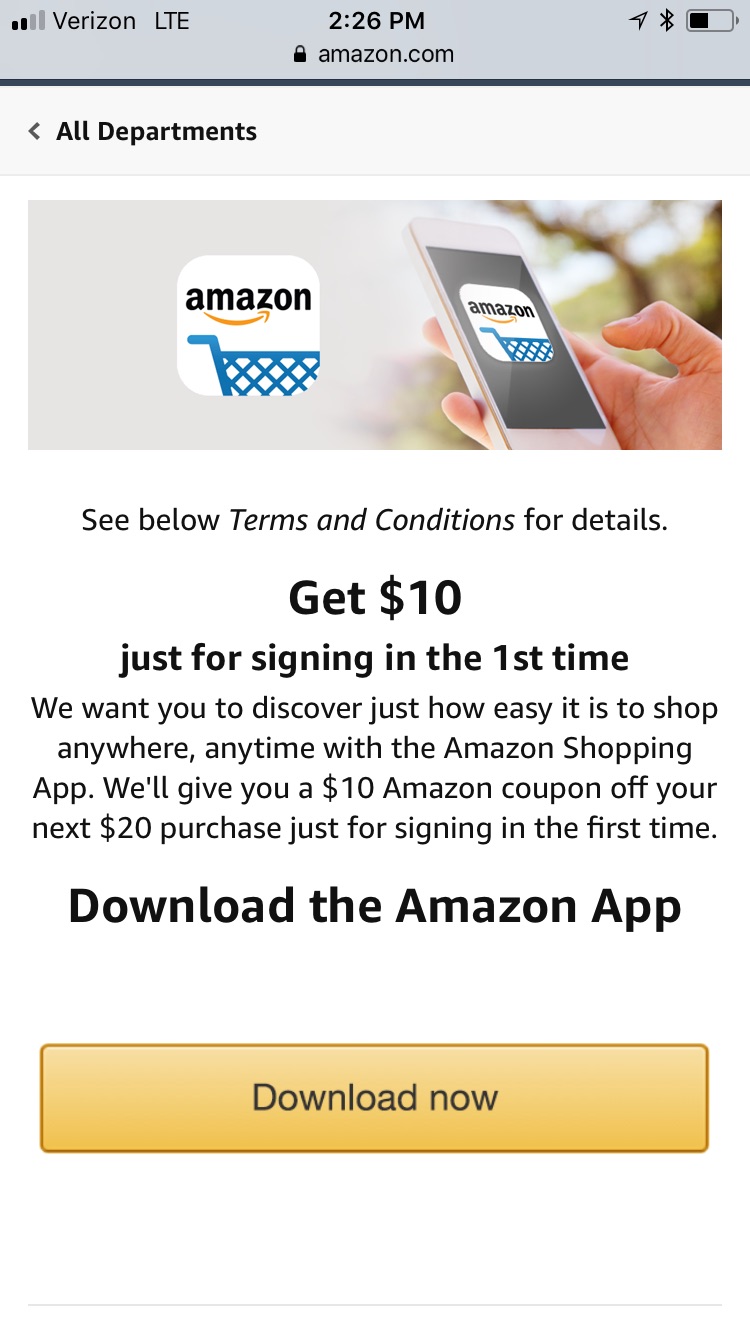The image depicts a screenshot of an Amazon.com promotion as viewed on a cell phone screen. In the top left corner, there is the Verizon network indicator followed by an LTE signal strength symbol. The current time displayed in the center is 2:26 p.m., while the top right corner shows a Bluetooth icon and a battery icon indicating it is about half full. 

Directly beneath these icons, "Amazon.com" is prominently displayed, followed by the dropdown menu for "All Departments." Below this header, the Amazon logo is visible alongside part of a blue shopping cart icon. The background of the screen is primarily grey with a faded image of a tree.

The main text reads: "See below terms and conditions for details. Get $10 just for signing in the first time. We want you to discover just how easy it is to shop anywhere, anytime with the Amazon shopping app. We’ll give you a $10 Amazon coupon off your next $20 purchase just for signing in the first time."

At the bottom, there is a prompt to "Download the Amazon app," accompanied by a yellow rectangle button labeled "Download now." The background of the promotional text and buttons is white, making the information stand out clearly.